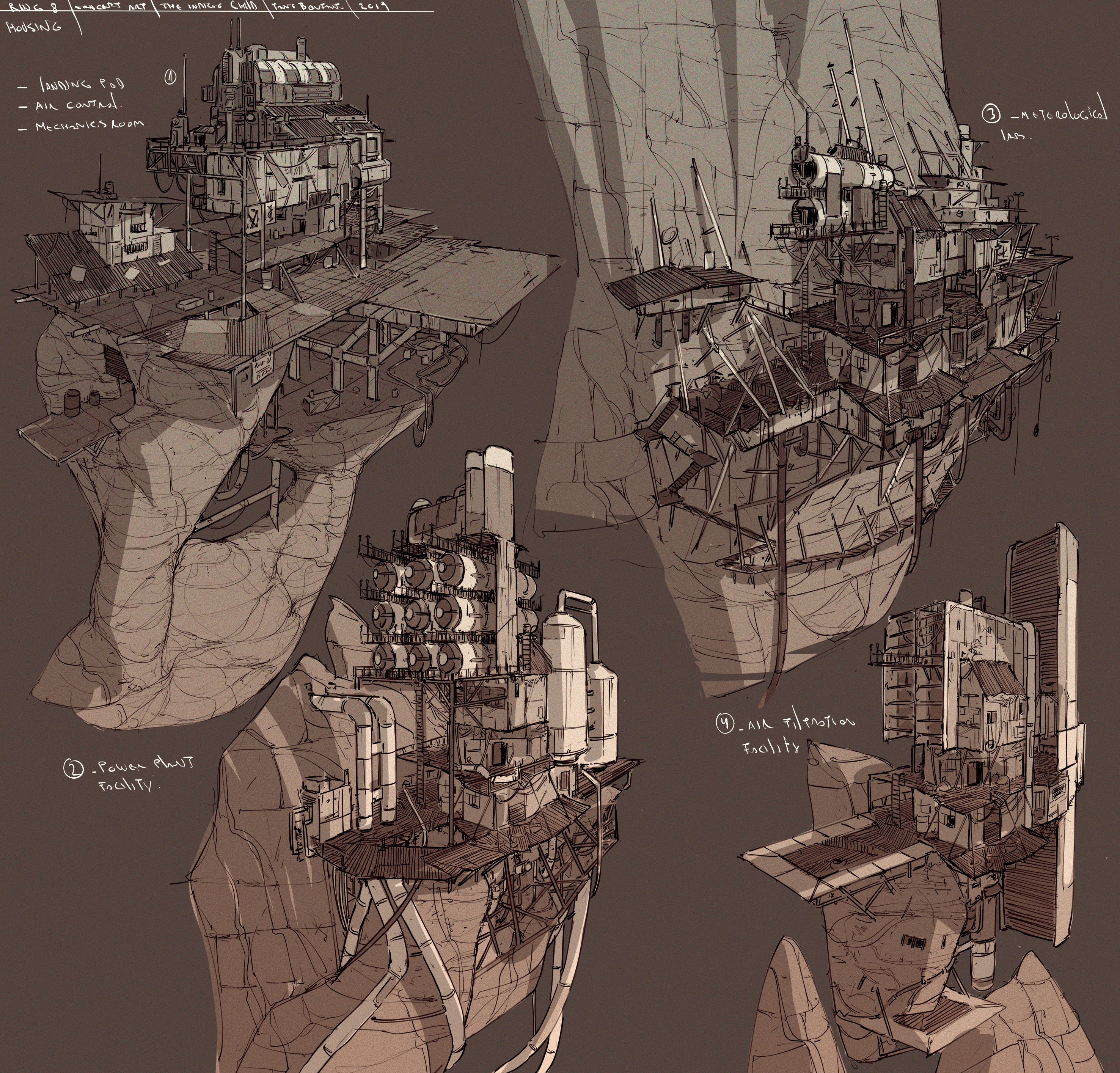The image is a detailed, artist's rendition done primarily in brown tones with some cream highlights. It features four intricate steampunk-style blueprints that depict an imaginative blend of industrial machinery and residential structures built into rocky cliffs or boulders. The drawings suggest a post-apocalyptic world reminiscent of scenes from films like *Waterworld* and *The Postman*. Each of the four segments shows a different configuration of these mechanical constructs: 

- The top left section illustrates a house with tanks on its roof, integrated with ladders and various signs.
- The bottom left segment shows an industrial facility attached to a mountaintop, complete with gas tanks, tubing, and oil barrels, hinting at energy production or resource extraction.
- The top right quadrant portrays a three-story house precariously perched on the side of a cliff, supported by wooden scaffolding and interconnected bridges.
- The bottom right part displays a smaller but similarly structured building also affixed to the cliffside.

Despite some illegible white scribbles on the image, the overall theme suggests these mechanical cities or facilities are designed to blend into natural rock formations, as if for protection or concealment, showcasing a vivid blend of function and dystopian style.